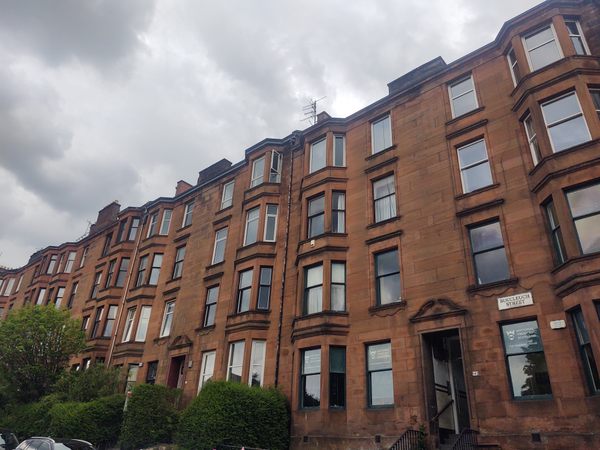This is a detailed photograph of several connected brownstone buildings, likely office or commercial properties, characterized by their light to medium brown large stones. The buildings are multi-level, with four stories and feature numerous architectural details, including pediments over the front doors. The photo captures dark-silled windows reflecting an overcast, cloudy sky. An old-style antenna, possibly a lightning rod, is visible on the dark gray or black roof. In the foreground, well-manicured green bushes and shrubbery are present, with the tops of a few cars partially visible. A street sign, with the legible word "street," indicates this is a city street, potentially in cities like Boston, potentially London due to the architectural style. The overall scene is devoid of people, emphasizing the quiet, dreary atmosphere of the overcast day.